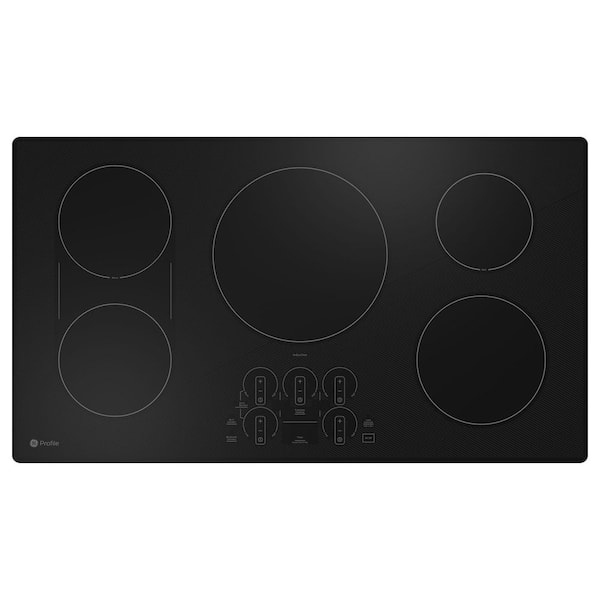The image depicts a rectangular, black surface featuring five circles outlined with thin, light-colored lines, resembling the layout of a stovetop. Dominating the center near the top is the largest circle, and positioned on the right side, there are two circles with the smaller one above the larger one. On the left side, two smaller and identical-sized circles appear, connected faintly by thin lines. Below the central circle, there is a panel with various touch controls, including plus and minus signs encircled with semicircles, possibly indicating battery-related functions. Despite the complex design, there are no other significant markings to clearly identify the exact purpose of the image. Additionally, a faint logo is located in the bottom left corner, further hinting at a specific device.